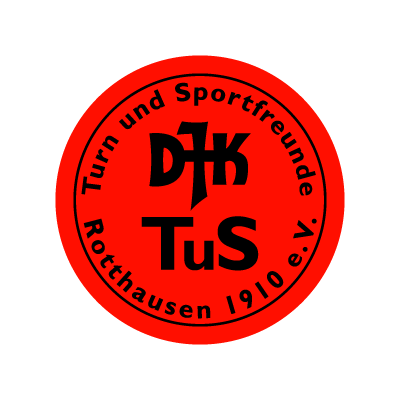This image features a distinctive red circular logo with a black inner ring close to the edge. The text within this black ring is German and arcs around the circle. At the top, it reads "Turn und Sportfreunde," while the bottom part of the circle says "Rathausen 1910 E.V." In the center of the logo, there are two lines of text with the top line displaying the letters "DTK," which appear to be stylized and connected, and the bottom line saying "TUS" with a lowercase "u." The black ring creates a clear boundary, providing contrast between the inner text and the red background, giving the logo an iconic and formal appearance. The design elements and German text suggest it might represent a historical or traditional German organization, likely established in 1910.